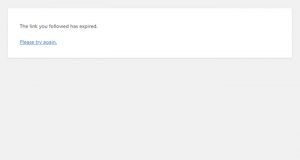The image displays a pop-up notification set against a light gray background. The pop-up itself is presented as a light gray rectangle, centered within the image. Near the top of this rectangle, there's a smaller white rectangular box containing text. 

On the left side of the white box, in black text, the message reads: "The link you followed has expired." Below this, a blue, underlined text reads: "Please try again," indicating it is a clickable button intended to reload the page.

Surrounding the white text box, very thin light gray lines border the top, left, and right edges, ensuring the white rectangle does not occupy the entire width of the gray pop-up. The lower half of the pop-up, extending downwards, remains blank, filled with the same light gray background, giving a clean and minimalist look to the notification.